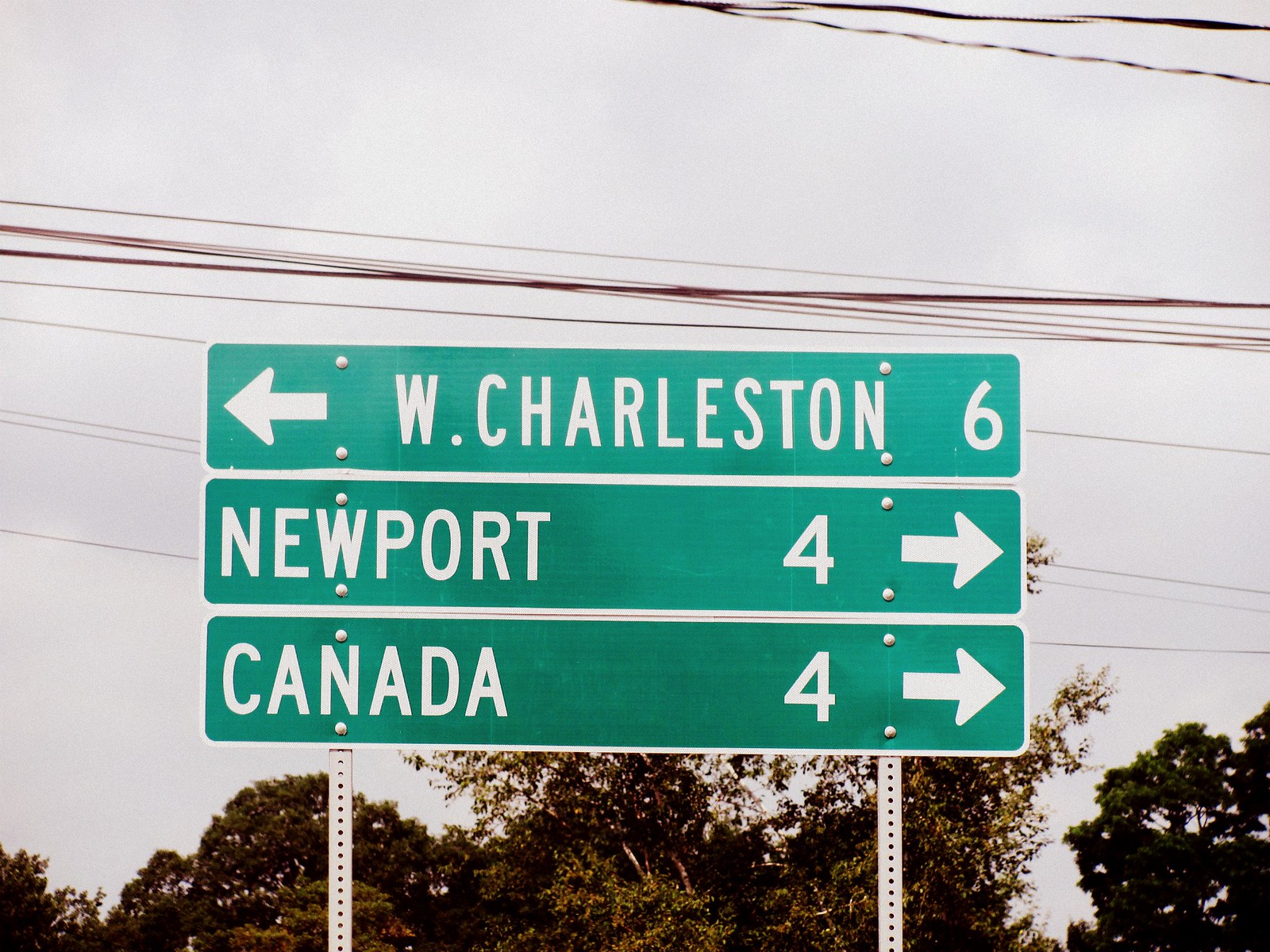The image features a green directional street sign fixed onto two light gray metal poles with perforations. The sign is divided into three horizontal sections. The top section directs to "W. Charleston" with a left-pointing arrow and the number "6" next to it, all in white text. The middle section reads "Newport" with a number "4" and a right-pointing arrow. The bottom section indicates "Canada" with a "4" and another right-pointing arrow. Surrounding the sign are dark green trees in the lower background, telephone wires running horizontally, and a light gray, overcast sky above.